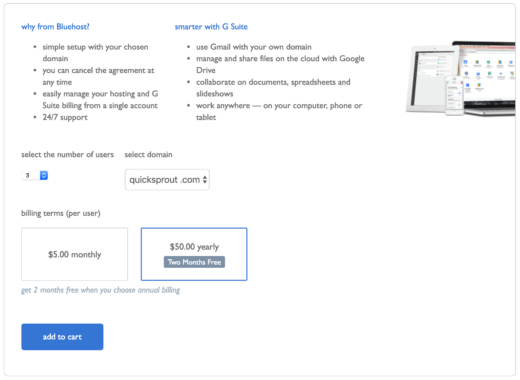The webpage, predominantly white in color, appears to be promoting services from Bluehost and G Suite. At the top, it prominently features questions prompting user engagement, suggesting it might be the second page of a flow or service setup process. The header spells out benefits with statements like "Why Bluehost?" and "Get Smarter with G Suite."

Below the introductory section, concise bulleted points in black provide further information about the services. Key points include:

- Simple setup with your chosen domain
- 24/7 support
- Option to cancel the agreement at any time

Next to these, under the "Smarter with Gmail" heading, the offerings include:

- Use Gmail with your own domain
- Manage and share files on the cloud with Google Drive

In the center of the page, there's a section where users can configure their service plan:
- A dropdown menu pre-filled with "three users"
- A domain field set to "quicksprout.com"
- Billing terms presented with two options: a white box for "$5 monthly" and a blue box for "$50 yearly" with a note indicating "two months free" with the annual billing option

A brief note below reiterates this deal, stating, "Get two months free when you choose annual billing." A blue button with white text reads "Add to Cart."

On the right side of the page, there is a visual displaying an iPad, an iPhone, and a laptop, all showcasing various icons on their screens, adding a tech-centric aesthetic to the webpage.